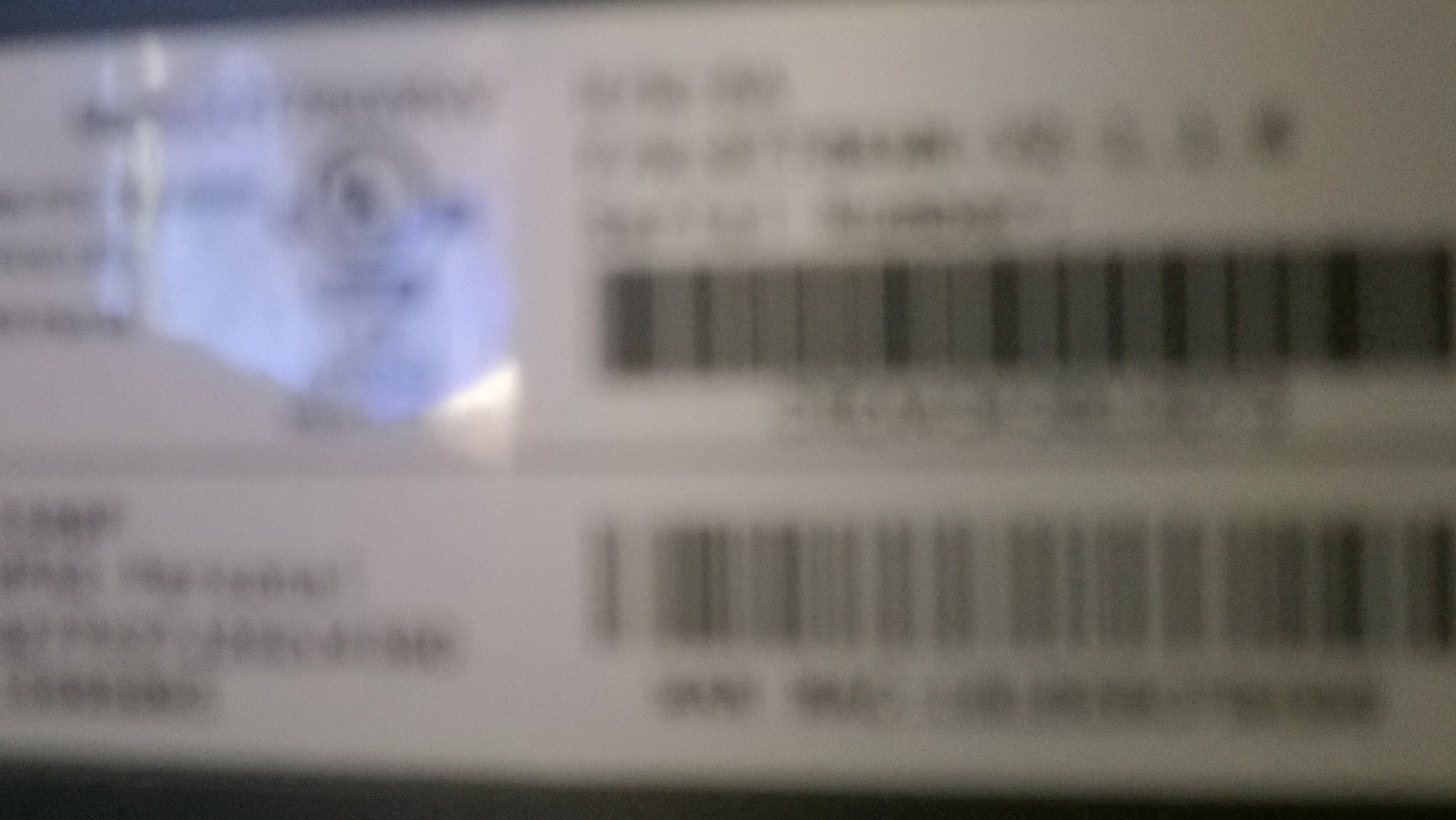Two wristbands are placed on a black surface, possibly a table or desk. The image is quite blurry, making it difficult to discern details. Each wristband features a distinct serial number, both of which are visible. Above the second wristband, there is some writing that is partially cut off from the view of the first wristband. Additional text is present to the left of the wristbands. The top wristband has an image resembling a fish with its mouth wide open, showcasing numerous teeth. The fish-like figure has large eyes positioned on the top of its face, giving it an almost amphibian, frog-like appearance.